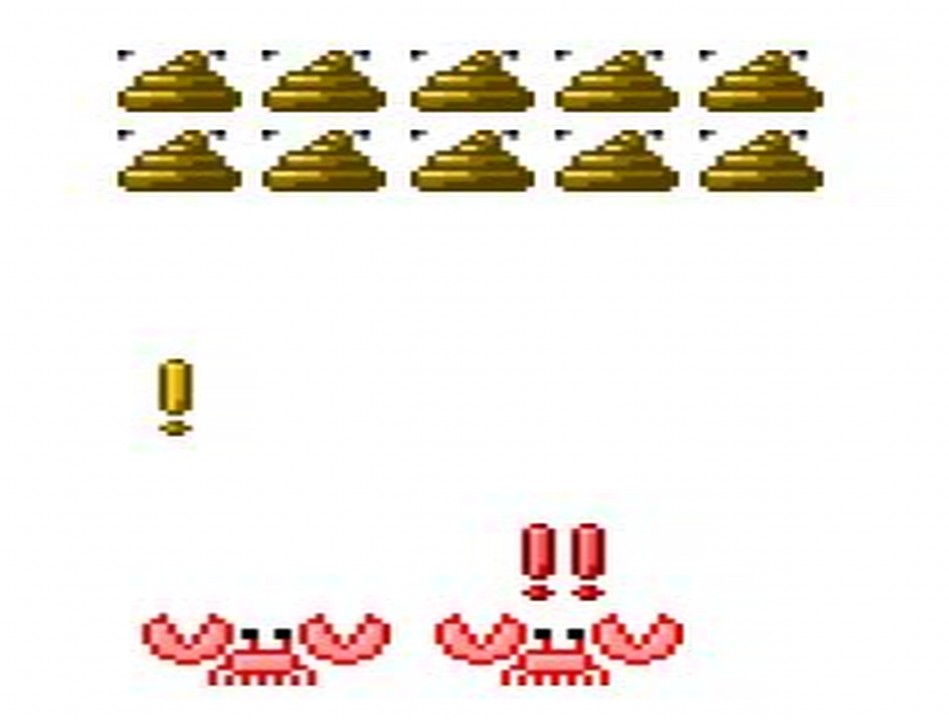This image showcases a scene from a retro-style, pixelated video game. At the top of the screen, there are two sets of five beehives, each adorned with black bee outlines in their top right and top left corners. These beehives are intricately designed with dark brown, green, and gold hues, giving them a vibrant yet vintage appearance. Below the beehives, a gold-colored, rectangular missile can be seen shooting upwards towards them. Further down, two highly pixelated pink crabs are centrally positioned, each with two open arms extended outward. Just above the lower right crab, two pink rectangular objects are directed upwards, seemingly aiming for the beehives as well. The meticulous pixel art and dynamic action elements create a compelling and nostalgic visual of classic arcade gameplay.